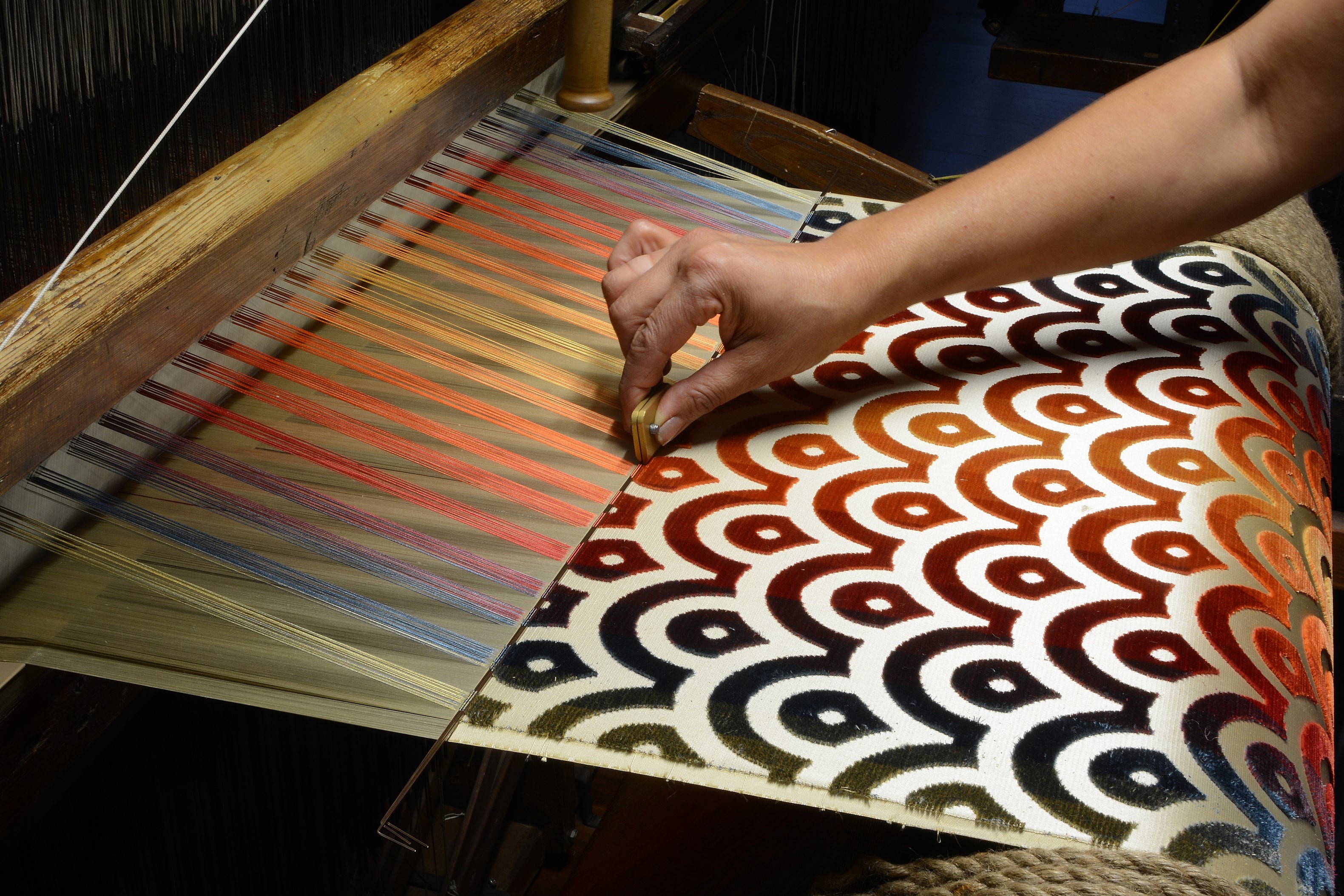A detailed and enriched description combining elements from the three captions:

The photograph captures an individual diligently working at a loom, with their arm extending from the top right corner and reaching towards the middle of the image. The primary focus is on the colorful textile being woven, which displays a striking gradient pattern. This pattern transitions smoothly from blue at both ends to yellow in the center, due to intertwining different colored threads, upon which multiple shades of blue, purple, red, orange, and green are present on the loom's left side.

The partially completed textile, featured prominently from the middle towards the right, exhibits a plush, bubbly texture reminiscent of the playful, geometric designs typical of the 1970s. Despite its simplicity, the textile's eye-catching gradient, combined with its silken appearance, suggests a substantial depth and intricacy.

Additional visual interest is provided by the wooden frame of the loom, visible at its top, and the various threads and ropes positioned in the bottom right corner. The lighting is entirely artificial, emanating from a source directly above, casting a focused illumination on the loom and enhancing the texture and vibrant colors without revealing any background elements beyond the loom and the person’s arm.